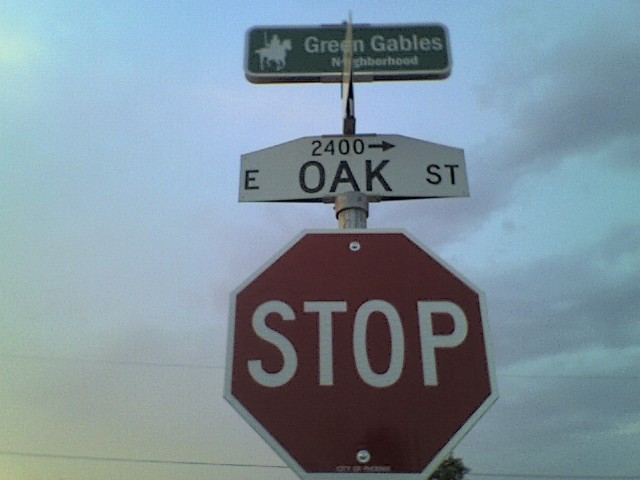Caption: 

In the foreground stands a typical red stop sign with bold white letters reading "STOP." Attached to the same post are three additional signs. Directly below the stop sign, a small rectangular sign reads "City of [unreadable]." Above the stop sign, another rectangular black and white sign denotes "East Oak Street" and the number "2400," indicating the address of the 2400 block of East Oak Street. This sign includes an arrow pointing to the right. The highest sign displays "Green Gables Neighborhood" in white text against a green background, accompanied by an illustration of a knight riding a horse to the left of the text. The backdrop features a cloudy sky with a few electrical cables running horizontally, akin to telephone lines.